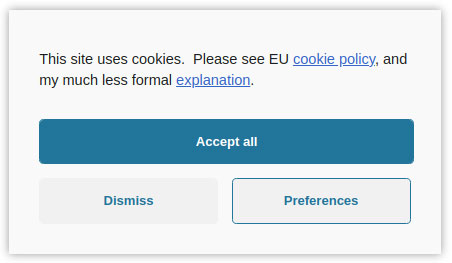In the image, there is a pop-up box commonly seen on websites regarding cookie policies. The box has a subtle shadow or shading around its edges, which gives it a slightly elevated appearance against the white background. At the top of the box, there is black text that reads: "This site uses cookies. Please see our EU Cookie Policy, and my much less formal explanation." Both phrases "Cookie Policy" and "explanation" are underlined in blue, indicating they are clickable hyperlinks that will redirect the user to other pages for more information.

Below this text, there is a prominent turquoise blue button with white text that reads "Accept All." Beneath this button, there are two additional buttons. The first is a white button with blue text that says "Dismiss," and the second is a white button with a blue border that says "Preferences," suggesting it is the currently selected option.